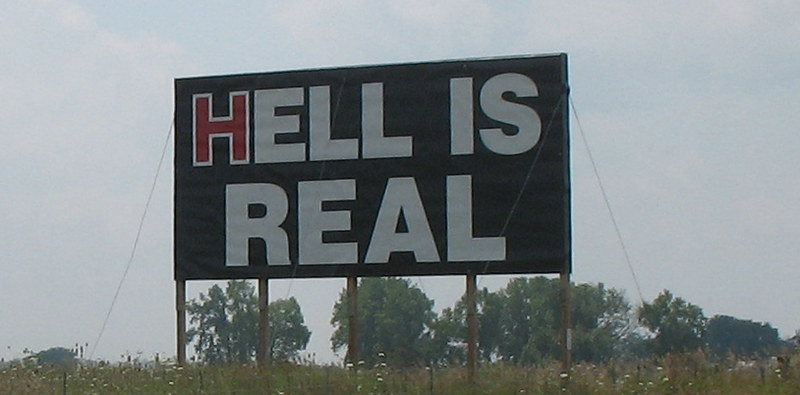The image depicts a large billboard prominently placed perhaps alongside an interstate or major highway. The billboard is supported by five sturdy brown poles and further secured by guide wires extending from the end poles. The sign itself has a stark black background with bold, white text that reads "HELL IS REAL," with the "H" standing out in red. The setting is an expansive grassland with tall green grasses and interspersed wildflowers. In the background, there are scattered trees and a small building, with the sky above being a light blue speckled with some clouds.